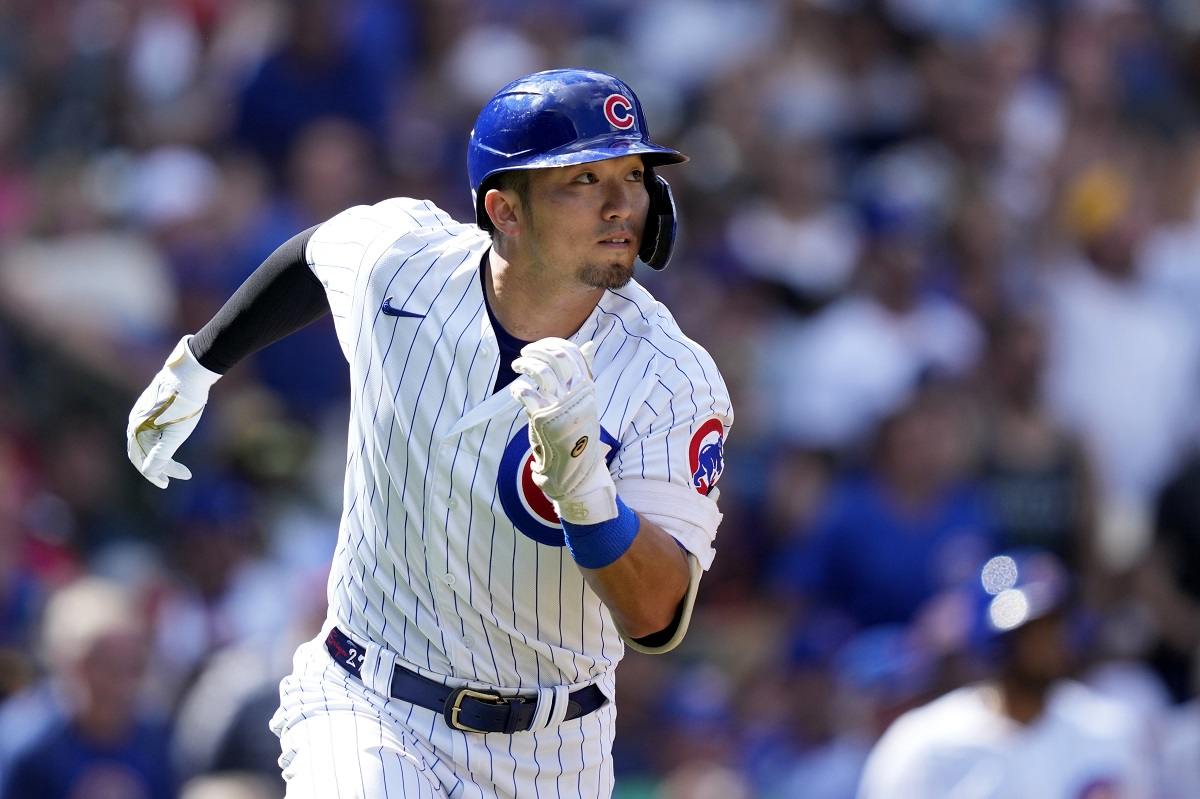In this vibrant action shot, a Chicago Cubs baseball player is the focal point, positioned slightly to the left of the frame. He is mid-stride, appearing to run towards first base, his gaze fixed on the distance, likely tracking the flight of the ball he just hit. The player dons the iconic Cubs uniform, featuring white with blue pinstripes and a distinctive large 'C' logo in blue and red on the left side of the jersey. A Nike symbol is prominent on the right side of his chest. His ensemble includes white batting gloves, a blue compression sleeve on his left arm, and a black belt secured around his waist. Atop his head is a bright blue helmet with the signature red 'C' logo, a mark of Chicago pride. The backdrop reveals a crowd of fans in the bleachers, adorned in blue and white attire, their indistinct forms and colors creating a dynamic yet supportive backdrop for the player. This professional photograph captures the intensity and movement of the game, resonating with the thrill of this moment in play.